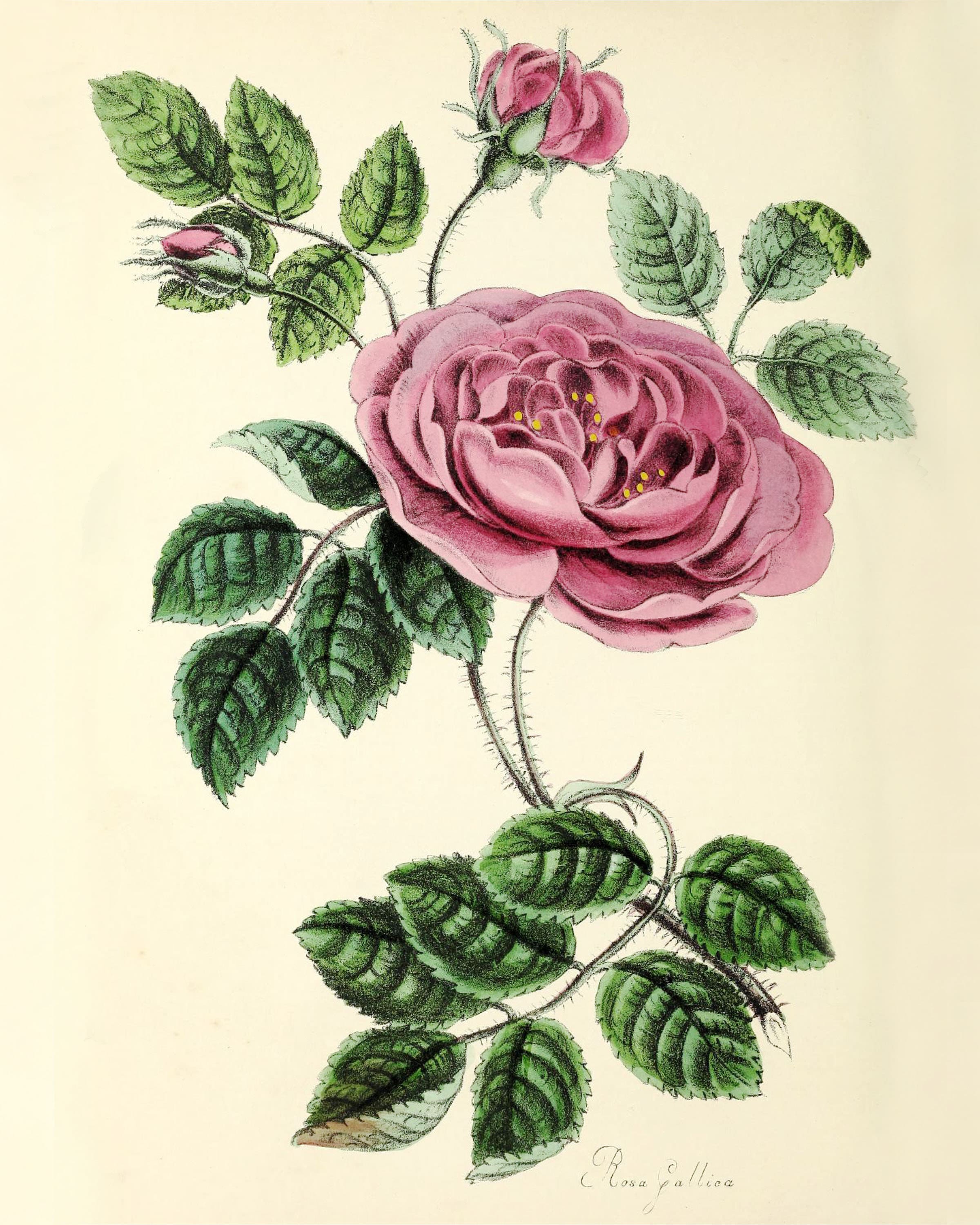This botanical illustration depicts a rose with three flowers in various stages of development, all set against a tannish yellow background. The central focus is a pinkish-purple rose in full bloom, exuding a muted, delicate charm reminiscent of Norman Rockwell's style. Surrounding the main bloom are leaves branching out from five distinct stems, each leaf comprising an odd number of leaflets, typically three, five, or seven. 

Accompanying the fully open rose is a partially opened bud, showcasing some internal petals, and a small, tightly-closed bud with only its outer petals visible. The green leaves add a vibrant contrast to the pinkish hue of the flowers and extend outward from multiple directions. Thorny stems contribute to the authenticity and detail of the print. 

The bottom of the canvas bears the inscription "Rosa gallia," presumably identifying the genus and species of the rose. This composition captures the elegant evolution of the rose's blooming process, from bud to full blossom, all framed in a naturalistic, softly colored setting.